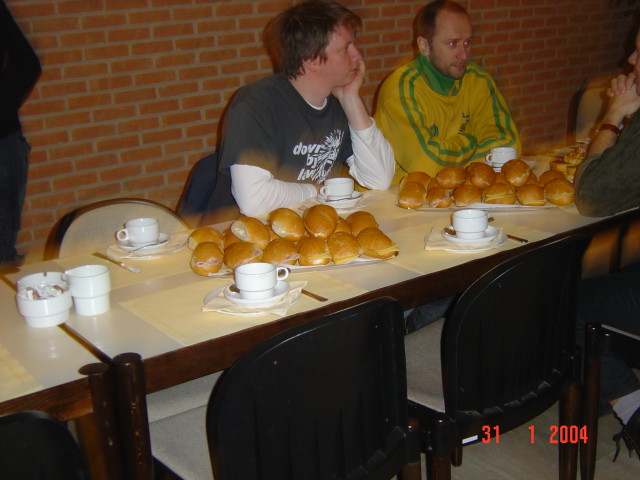This angled indoor photo captures two men seated at a small, narrow, white plastic-topped table with wooden edges and legs, which appears to be made up of several tables pushed together. The table is set under a red brick wall with white mortar. Each place setting includes a coffee cup and a saucer. On the left corner of the table sits an ashtray beside a small round white object. Two giant platters of golden-brown rolls are prominently displayed; one platter is located to the left of the first man, while the second is directly in front of him. The first man, wearing a gray t-shirt with a long white-sleeve shirt underneath, sits with his face in his palm, looking at someone across the table. To his right, the second man wears a green and yellow sports jersey with a zippered collar, observing the scene to his right. In the far-right corner of the image, an arm belonging to another man, who is wearing a wristwatch, is subtly visible. This third man appears to be seated across from the two main subjects. The bottom left of the photo features a timestamp, reading "31 1 2004."